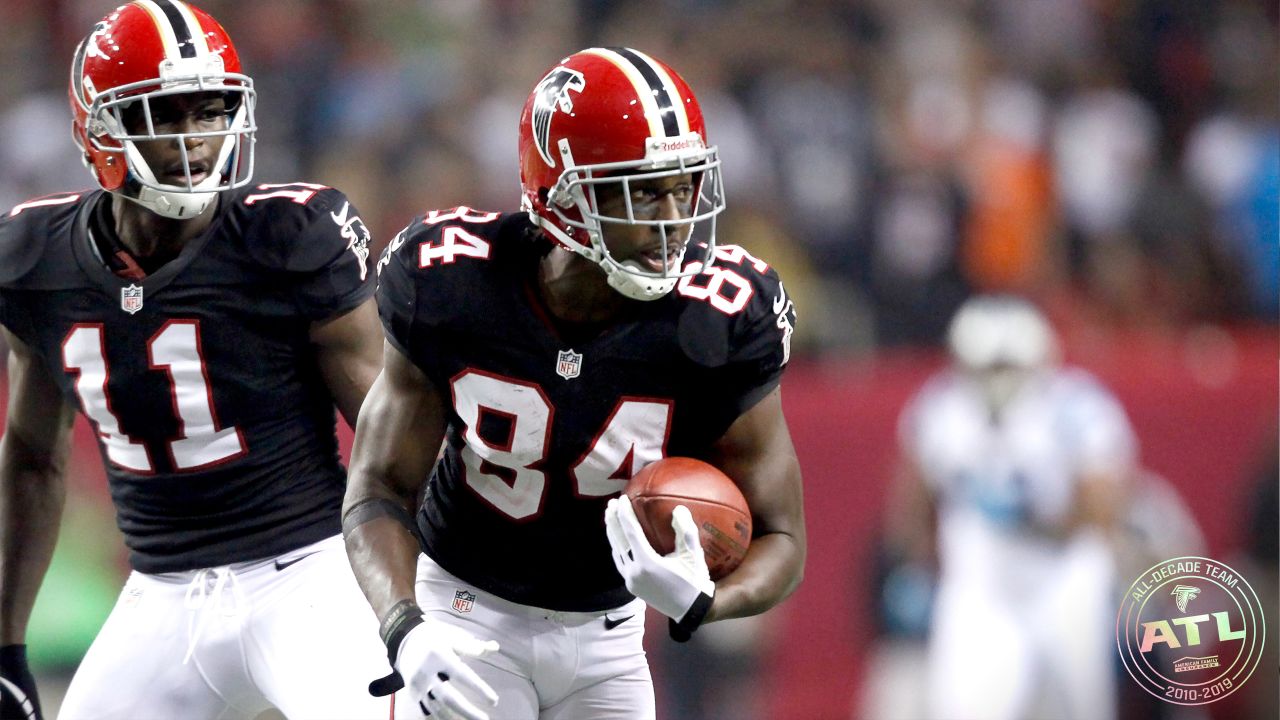In this vivid and bright photograph of an American football game, two prominent players of the Atlanta Falcons, identifiable by their dark blue jerseys with red outlines around white numbers, take center stage. On the left, player number 11, wearing a red helmet with a white and black stripe, stands focused, while on the right, player number 84 grips a football in his white-gloved hands, looking to his right and showcasing a tattoo on his arm. Both players are dressed in white pants displaying the Nike and NFL logos. The blurred background reveals a bustling crowd and what appears to be a coach giving directions, as well as an opposing player in an all-white uniform. In the bottom right corner of the image, a circular logo reads "All Decade Team" at the top, "ATL" in the center, and "2010-2019" at the bottom, accompanied by a somewhat indistinguishable mascot.